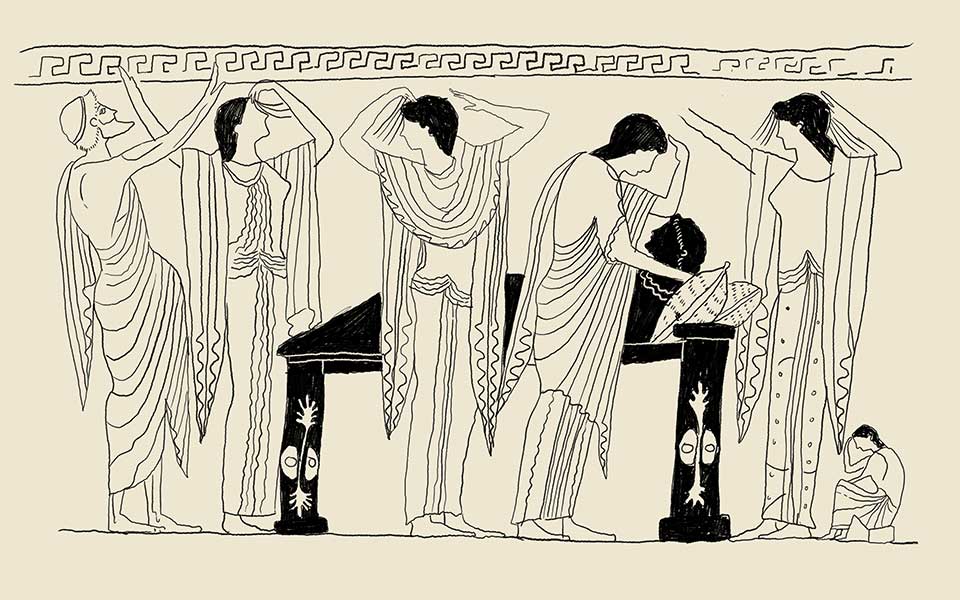This intricate black-and-white ink drawing, evocative of Egyptian art, features a procession of five prominently positioned figures clad in togas or long robes, each displaying distinct postures and gestures. At the uppermost part of the image, a Greek key pattern runs horizontally, accentuating the classical theme. On close observation, the first figure, a man wearing a toga and a skull cap, raises his arm up purposefully. Next to him, a woman with long hair and a toga wrap raises both arms skyward. The third figure, another woman with short dark hair, is adorned in a gown-like skirt and scarf and mirrors the dual arm-raising gesture. The fourth woman, similarly dressed with a toga and wrap, has one arm elevated while the other rests downward. The final tall figure maintains her toga and wrap with a smaller figure beneath her, arguably in a state of introspection, seated on a rock with her head in her hand.

In the background, atop a high table or raised bed, lies a shadowy figure, fully rendered in black, with pillows supporting their upper body. This striking figure appears to be the focus of collective grief, with the surrounding individuals, including the small seated figure, expressing various states of mourning. The contrasting black and white elements underscore the somber atmosphere, suggesting a scene laden with historical and emotional depth.